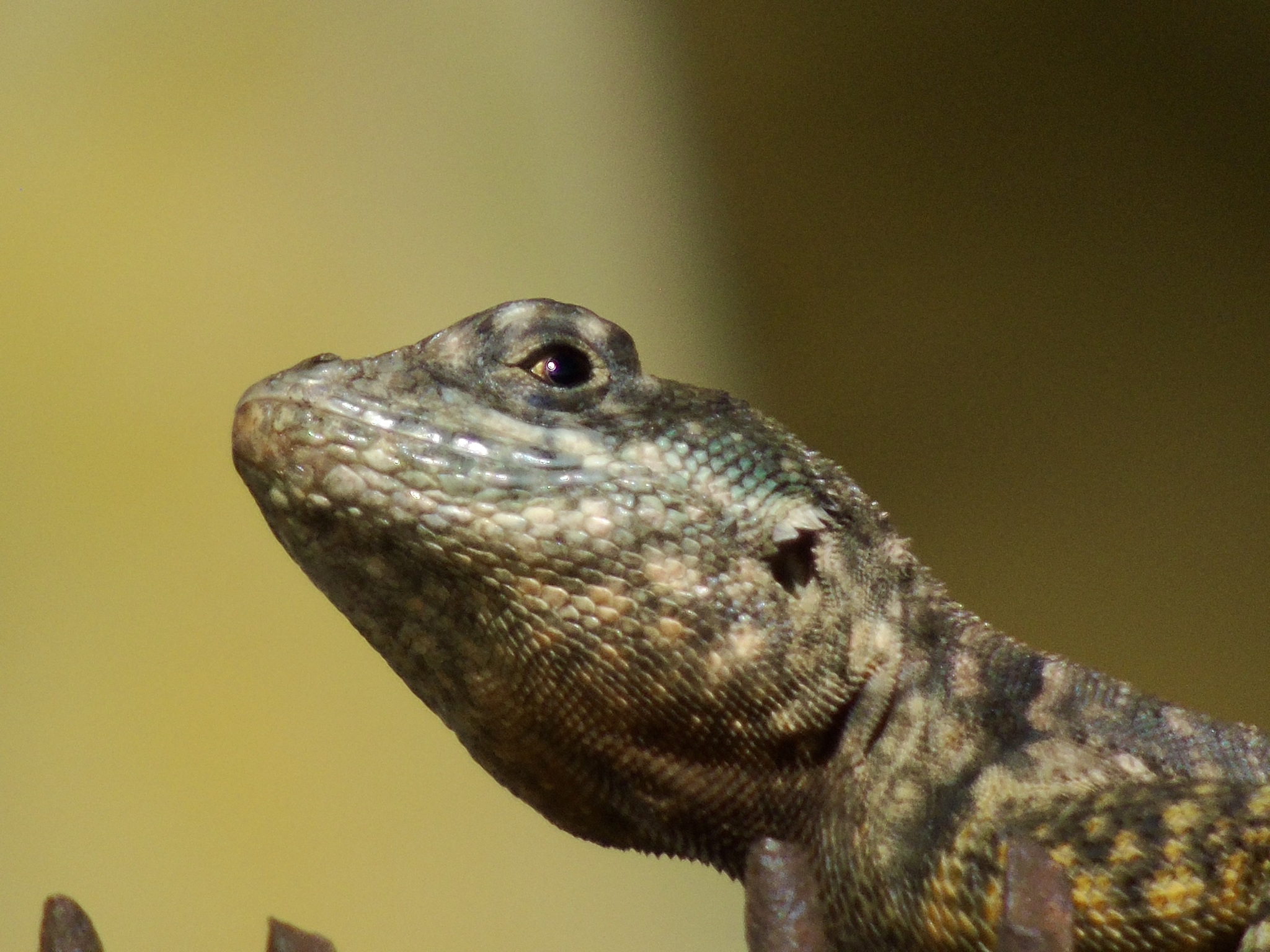This close-up photograph captures the head and neck of a lizard, possibly an iguana, presented against a blurred gradient background ranging from light green to dark brown. The high resolution details clearly showcase the lizard’s intricate scales, which are predominantly light green, medium green, yellow, and brown with specks of black, contributing to a natural camouflage appearance. The lizard's skin features a distinct pattern of spotted scales, blending brown, yellow, and cream hues especially around the neck area. The creature has an expressive face, with prominent ridges over its brown eyes, which also contain hints of pale yellow and exhibit a reflective white spot. The eye appears to be looking slightly off-screen, to the left. The lizard's mouth is closed, and it seems to be in a content demeanor, possibly peering over a small metal divider. The lizard's head and the top of its shoulders are centered in the image, with the head lifted, giving a slightly upward gaze. Overall, the photograph beautifully illustrates the detailed texture and coloration of the lizard’s scales and provides a glimpse into its serene and observant nature.